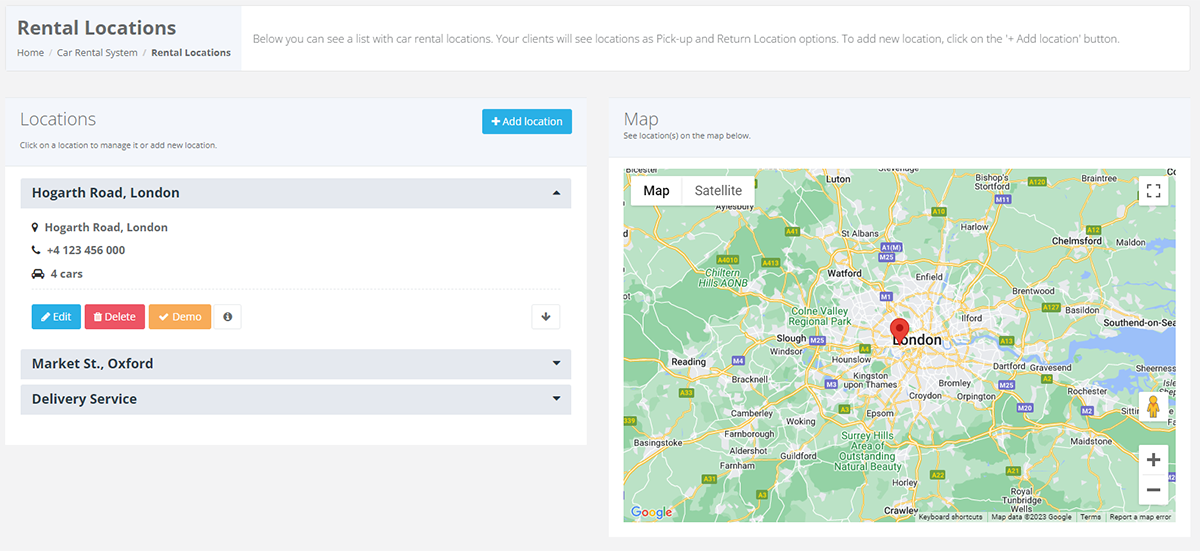The image depicts an interface for a car rental system. 

At the top left, there is a small rectangular section with a light gray background featuring a bold gray font header that reads "Rental Locations." Beneath this header is a menu divided by spaces and forward slashes. The menu options, listed in gray, include "Home," "Car Rental System," and "Rental Locations." The "Rental Locations" option is highlighted in bold, indicating it is the currently selected option.

On the right-hand side of the image, there is a long rectangular section with a white background and small gray text. It states: "Below, you can see a list with car rental locations. Your clients will see locations as pickup and return location options. To add a new location, click the plus add location button." 

Below this, the interface transitions to a light gray background. On the left, within a rectangular area that has a bluish tint, is a section headed "Locations." Beneath this, small black letters instruct the user to "Click on a location to manage it or add a new location." 

In the top right corner of this section, there is a rectangular button with a blue background. This button features a bold white checkmark on the left side and non-bold white text that reads "Add Location."

Further down, the interface displays a white background rectangle. At the top of this rectangle, there is a header with a gray background and bold black text that reads "Hogarth Road, London." Directly beneath this header, there is a small gray map pin icon followed by the text "Hogarth Road, London."